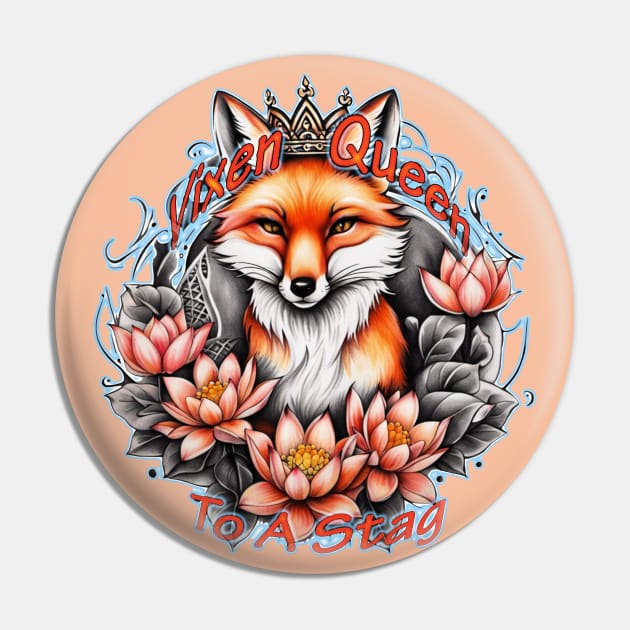The image in front of me is a square, full-color photograph set against a gray background, showcasing a round illustration. Dominating the center is a fox rendered in earthy tones of white and burnt orange. This regal fox is adorned with a crown, reinforcing its majestic persona. Encircling the fox are vibrant pink orchids with yellow centers, their leaves depicted in shades of gray. The entire composition has a distinctive graffiti or street art style, accentuated by blue graffiti elements along the outskirts of the image. The text "Vixen Queen" is prominently displayed at the top in a burnt orange hue, while "to a stag" is inscribed at the bottom in the same color. The circular illustration might be on an object such as a frisbee or a pin, with the unillustrated portions bathed in a pale pink pastel shade.